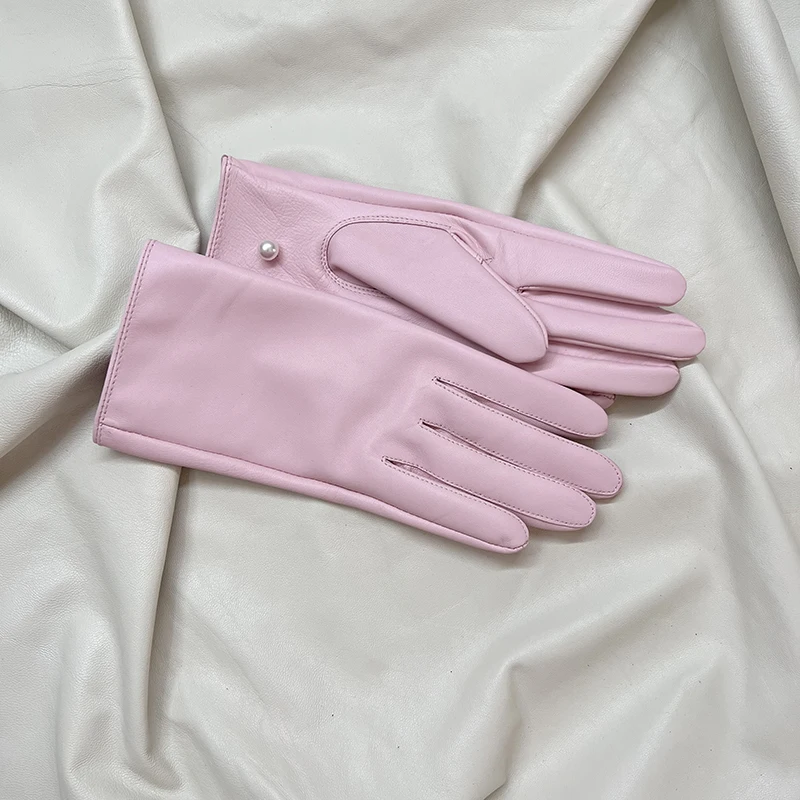A meticulously arranged bird's-eye view photograph features a pair of chic, light bubblegum pink leather gloves elegantly displayed on a silky, folded white or cream sheet that serves as the background. The background's texture is reminiscent of draped leather, adding a seamless continuity with the gloves. The right glove is placed palm down, showcasing the top side with detailed hemming along the fingers and wrist. In contrast, the left glove faces upward, partially tucked beneath the right, revealing an exquisite, small, shiny white pearl embellishment near the thumb. The photograph's soft lighting accentuates the feminine and sophisticated nature of the scene, making it ideal for a high-end product ad.